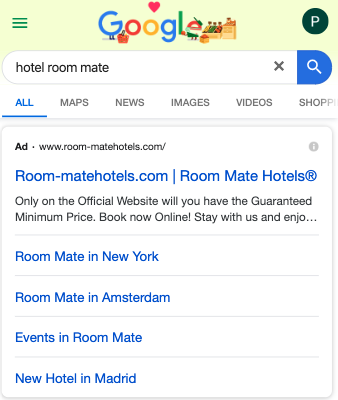A person is conducting a Google search on a festive-themed day, possibly Valentine's Day or Mother's Day, as indicated by Google's special doodle. The doodle features a pink heart over the second yellow 'o' in the Google logo, with additional elements suggesting a celebration, such as a bird and several animated characters. Notably, the blue 'G' has legs on the left, and the 'E' appears to be wearing a green hat. The usual three horizontal lines indicating a menu are present but are green instead of black.

The search bar is oval with a light gray outline. The user has entered the search term "hotel room mate," with a space between "room" and "mate." To the right of the search query, there is a bold gray 'X' for clearing the search. The right end of the search bar transitions into a blue section with a white magnifying glass icon in the center.

Below the search bar are tabs for different search categories – All, Maps, News, Images, Videos, and Shopping – although "Shopping" is partially obscured. The 'All' tab is selected, indicated by its bold blue text and underline. The page's main content area is lightly gray, overlain by an advertisement.

This ad is contained within a square box with rounded corners and a subtle gray shadowed border. At the top left of this ad, in small bold black text, is "Ad," followed by a black bullet point and further text reading "www.room-matehotels.com/".